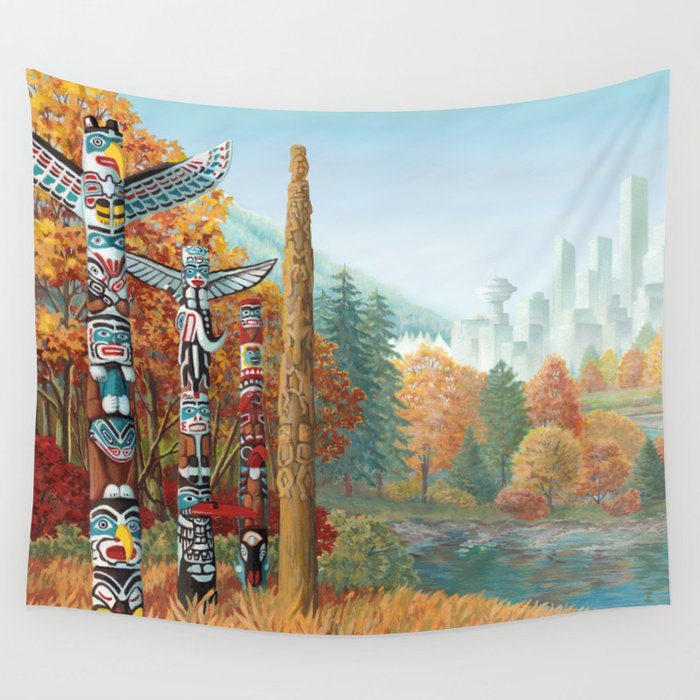The image showcases a richly detailed scene depicted on a fabric, possibly an oil or acrylic banner, hanging on a wall and partly cascading down in the middle. On the left side of the fabric, there are four totem poles intricately carved with traditional native patterns. Three totem poles are vibrantly painted, featuring a mixture of creature and human forms, two of which have wings. The fourth totem pole remains unfinished, displaying bare wood at the bottom. Moving to the center of the scene, a stunning autumnal forest emerges, with a vivid palette of red, orange, and yellow hues signaling the fall season. The forest is composed of a mix of spruce, pine, and maple trees. Further in the distance, a serene body of water, possibly a lake or river, lies adjacently. The background is dominated by a futuristic cityscape, with tall, gray high-rise buildings set against a clear blue sky, creating a striking contrast between past traditions and modern development. The foreground grass, reminiscent of a wheat field with shades of orange and yellow, enhances the depiction of the autumn setting.